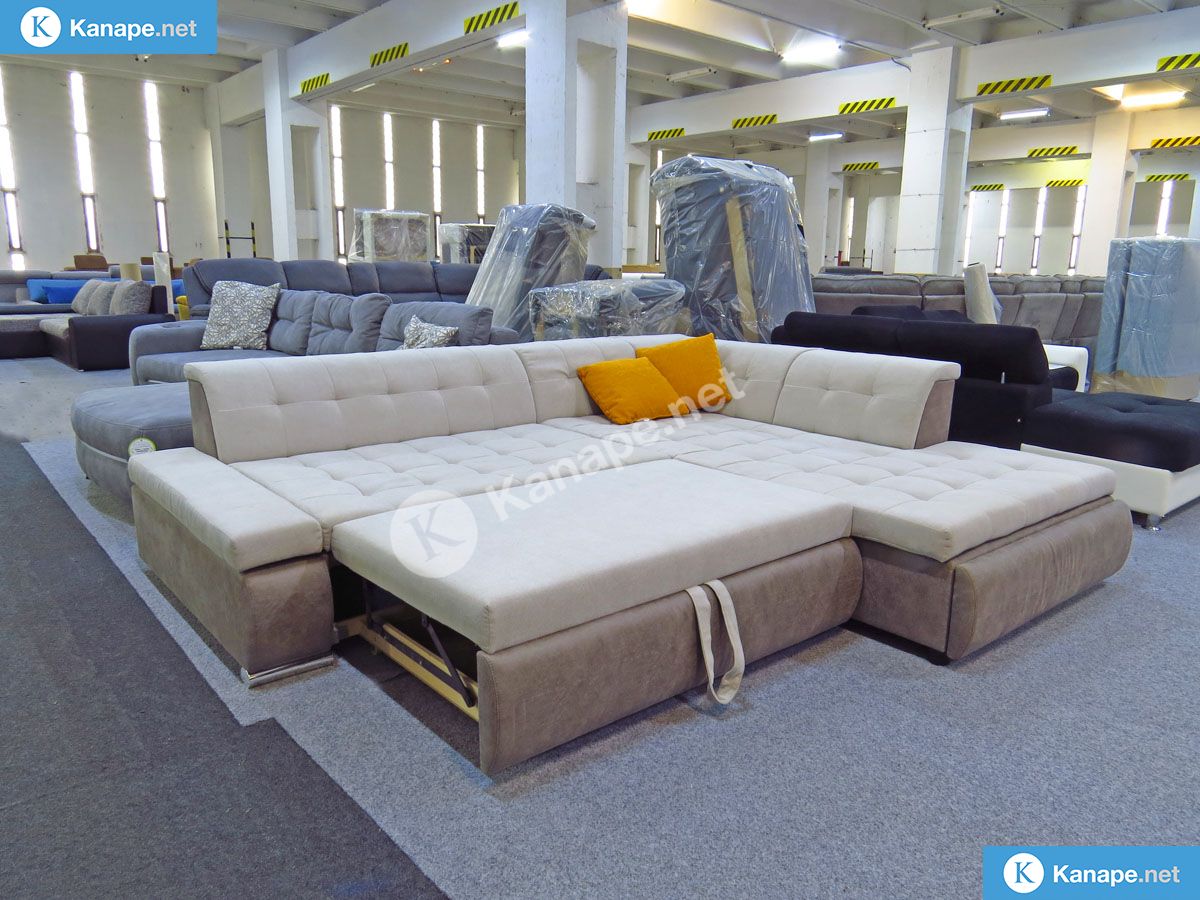The image depicts a large, industrial-style furniture showroom associated with Canapay.net, as indicated by a blue label situated in the top left corner. The showroom is an expansive open space with white walls and supporting columns, some of which are striped with yellow and black patterns, adding a decorative touch. Overhead, long linear lights illuminate the area. It is filled with an assortment of couches and sectionals in various pastel shades like blue, beige, gray, and some wrapped in plastic. The centerpiece of the image is a tan, L-shaped sectional couch with plush, pillow-like cushions adorned with buttons, suggesting a blend of comfort and style. Surrounding it, various other pieces, including a black and white sectional and multiple blue couches, reflect the diverse options available in this expansive warehouse. The overall ambiance gives off a structured yet inviting vibe, filled with an array of comfortable and cozy seating solutions.